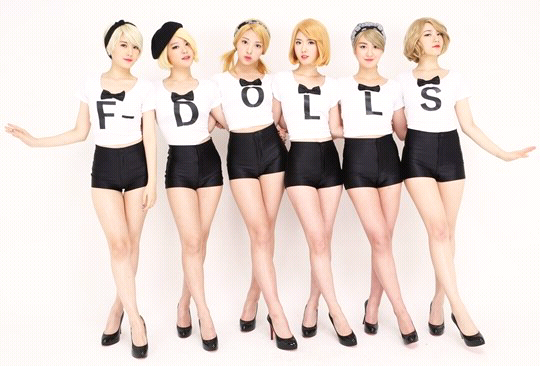The image depicts six young Asian women standing against a white background, all dressed in coordinated outfits. Each woman wears a white short-sleeved top with a black bowtie printed at the neckline, paired with high-waisted black shorts that show off their legs, and black high-heeled shoes. Their hair is shoulder-length or slightly shorter, light brown to blonde, and styled neatly. Notably, the woman second from the left sports a black hat, while the woman on the far right wears a black bandana. Their poses are uniform, with each woman crossing her right leg in front of the left and the ones in the middle placing their arms around their neighbors. The women on the ends have one arm extended outward. Each top is marked with large, black letters spelling out "F-D-O-L-L-S" across the group, presumably the name "F-Dolls." The attire, pose, and coordinated stance suggest they might be dancers or part of a performance group.